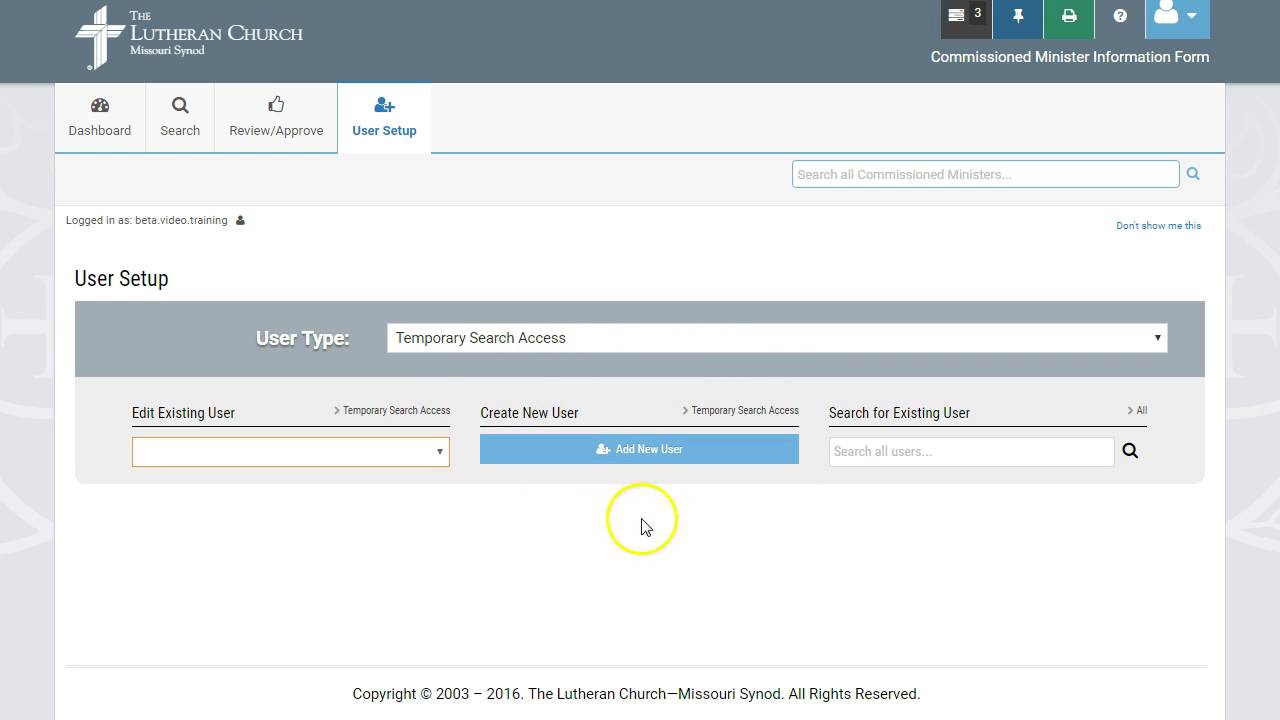The image appears to be a screenshot of an administrative dashboard for a Lutheran Church, specifically the Missouri Synod. The interface is framed by a dark gray border at the top and light gray borders on the sides, with a predominantly white central area interspersed with various shades of gray.

In the upper left corner, there's a prominent white cross accompanied by text in white that reads "The Lutheran Church, Missouri Synod." Below this header, a series of navigation boxes are visible with the labels: "Dashboard," "Search," "Review and Approve," followed by a highlighted blue box marked "User Setup," indicating that this section has been selected.

The main content area is under the "User Setup" heading, which is displayed in black text within a white background. Below this header, a large gray bar labeled "User Type" is followed by a white input field designated for "Temporary Search Access."

Further down, a lighter gray section contains options for user management, including "Edit Existing User," with an adjacent white input box, as well as "Create New User." Below this is a prominent blue box labeled "Add New User." There is also a designated area towards the lower right for "Search for Existing User," featuring another white input box.

Notably, a yellow circle with an arrow points towards the "Add New User" section, drawing attention to this feature.

At the very bottom of the interface, legal information is displayed, stating "Copyright 2003 to 2016, the Lutheran Church, Missouri Synod, All Rights Reserved."